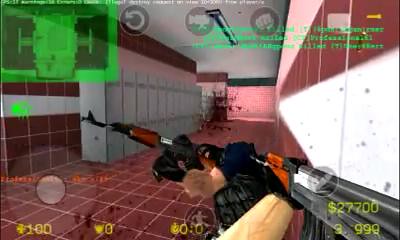This image depicts a gameplay scene captured with low-quality resolution, resulting in a blurry, pixelated, and fuzzy appearance. The image is uniquely shaped like a triangle. At the center of the image, there is a character holding a gun, which is colored brown and black. Towards the bottom right, there is another visible arm holding a gun. Additionally, in the bottom right corner, a money symbol can be seen, accompanied by the number "9999" below it. Despite the poor quality, the image conveys the elements typical of an action-packed gaming scenario.